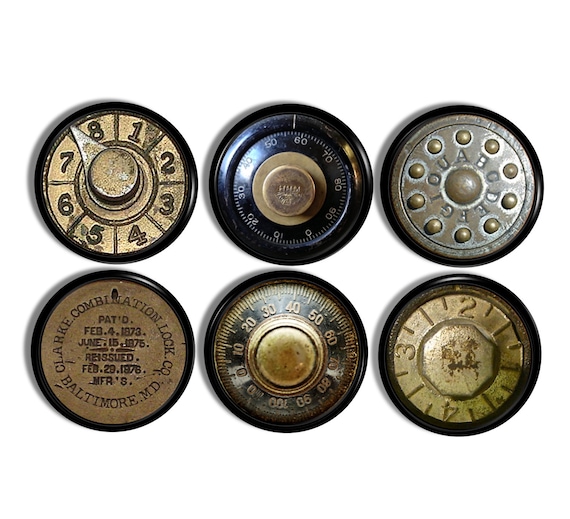The photographic image features six distinct dials arranged in two rows of three. Each dial is encircled with a black border. 

The top row of dials includes:
1. A dial labeled with numbers 1 through 8 and an arrow indicator.
2. A combination dial marked with increments from 0 to 90, resembling a traditional safe lock.
3. A dial displaying letters A, B, C, D, E, F, G, I, O, U.

The bottom row of dials features:
1. A dial inscribed with the text "Clock Combination Lock Company, Baltimore, Maryland, patented February 4th, 1873, June 15th, 1875, reissued February 29th, 1976, manufacturer."
2. A combination lock dial marked from 0 to 100.
3. A dial with numbers 1 through 4, separated by horizontal lines.

The arrangement and intricate details suggest a collection of historical and varied styles of combination locks.